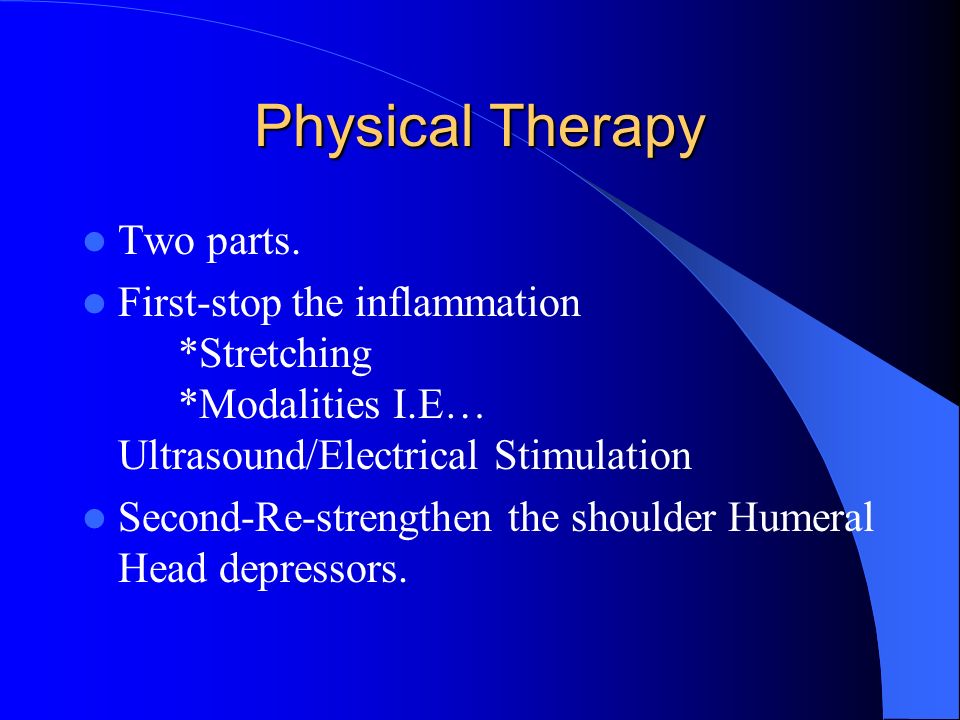The slide appears to be part of a medical educational presentation on Physical Therapy. The background is a gradient, transitioning from a bright blue on the left to a dark blue on the right. A ribbon graphic extends from the bottom right, starting thick and thinning as it moves to the top left. The title "Physical Therapy" is prominently displayed at the top in a light orange or pale yellow font. The slide contains three bullet points, all in white font with pale blue circular bullets. The first bullet point reads, "Two parts." The second bullet point outlines the first part: "First - stop the inflammation," followed by asterisks indicating subpoints such as "stretching" and "modalities (i.e., ultrasound/electrical stimulation)." The final bullet point states, "Second - re-strengthen the shoulder humeral head depressors." The layout is clean, well-spaced, and centered, typical of an educational PowerPoint presentation used in a medical setting.